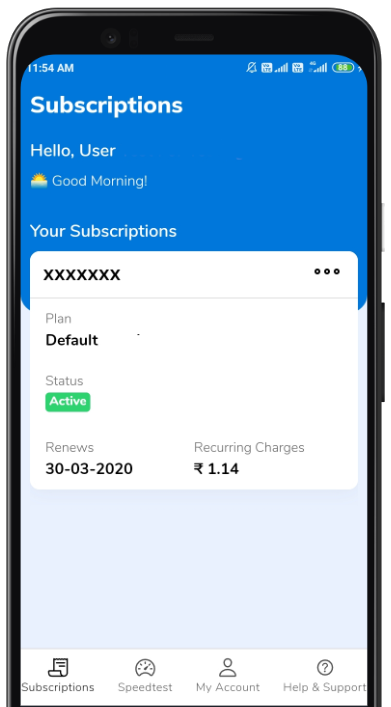The image depicts a smartphone screen displaying an application page. At the top left corner of the screen, the heading "Subscriptions" is written in white text against a blue background. Below this, a friendly greeting reads, "Hello, user. Good morning," accompanied by an illustration of a yellow rising sun.

Further down the screen, the section titled "Your Subscription" is shown. This section's text has a blue background, while the foreground displays the details in white. The subscription details are presented with placeholders "X's" for the subscription name. The subscription plan type is indicated as "default," and its status is marked as "active" with the word "active" highlighted in white on a green background.

The renewal information follows, stating that the subscription will renew on the 3rd of an unspecified month and year, for a recurring charge of 1.14 rupees. The bottom half of the app screen features a white background.

At the very bottom of the screen, four buttons or icons facilitate user navigation: 
1. The "Subscription" button with a page icon, written in black text.
2. The "Speed Test" button featuring a speedometer icon, in black text.
3. The "My Account" button with a person icon, in black text.
4. The "Help and Support" button with a question mark icon, in black text.

These icons are rendered in grey, and the descriptive text beside or beneath each icon is in black.